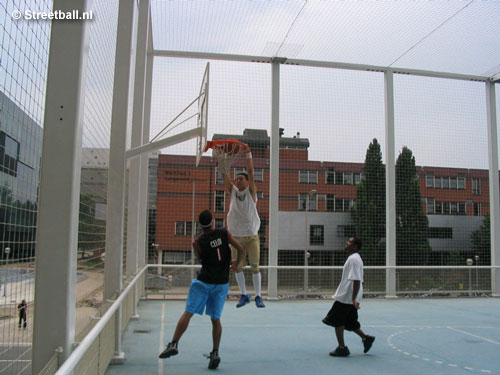This outdoor image, taken from streetball.nl in the Netherlands, captures a lively moment on a fenced basketball court with a light blue floor and white lines. The court is enclosed with a metal fence that even covers the ceiling, creating an outdoor room-like atmosphere. On the left-hand corner, there is a sign that reads "streetball.nl." The sky is mostly cloudy with hints of blue peeking through.

In the background, there's a prominent four-story brick building with numerous windows, possibly a school or office building, situated beside a smaller white-paneled structure reflecting the surrounding scenery. Further to the left, there's another building with a glass exterior. Two tall trees can be seen in front of the large brick building, and a sidewalk runs parallel to the buildings where a solitary figure walks in the distance.

On the basketball court, three men are engaged in a dynamic play. One man, who is dark-skinned, is wearing a black and partially red jersey with the number one, blue shorts, and black sneakers. Another man with lighter skin is performing a slam dunk, hanging onto the basketball hoop. He sports a sleeveless white tank top, khaki shorts, long white socks, and blue sneakers, with a wristband on his left wrist. The third player, also dark-skinned, watches the action from below, dressed in a white t-shirt, long black shorts, and black sneakers. The detailed composition of the players, buildings, and court creates a vivid and energetic scene.